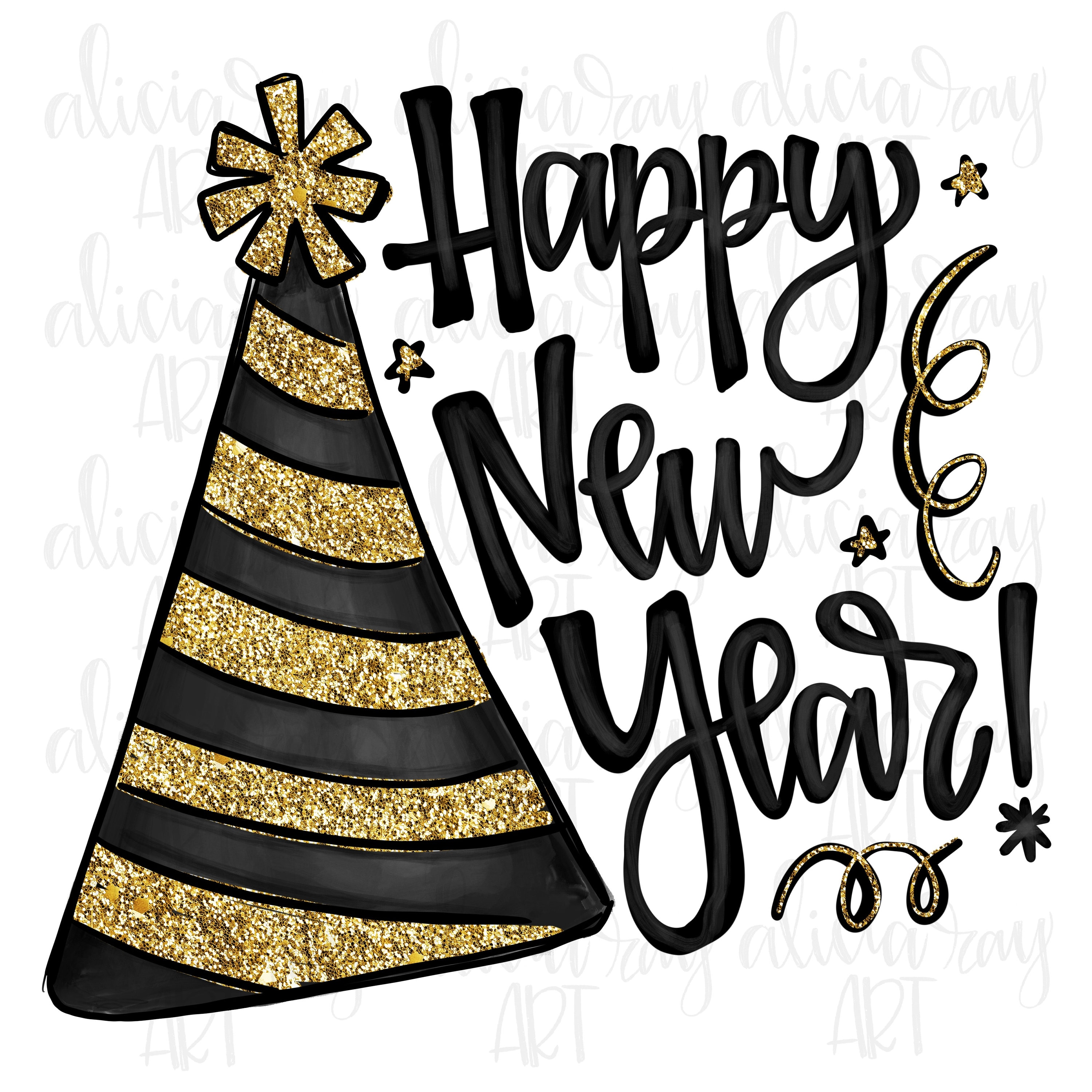This celebratory graphic is designed to capture the essence of New Year festivities and would be perfect for a banner, sign, or card. Dominating the design is the black, semi-cursive text that boldly announces "Happy New Year!" in a heavy script. To the left of this festive greeting is a striking party hat, shaped like a cone or dunce cap, adorned with alternating horizontal stripes of glittery gold and black. The party hat features a gold, asterisk-style star on top, adding to its festive appeal.

Surrounding the text and hat are swirls of gold glitter, stars, and confetti-like embellishments, enhancing the celebratory atmosphere. A very pale, almost watermark-like text in the background reads "Alicia," possibly indicating the artist's signature. This harmonious blend of elements creates a vivid and joyful image, perfect for ringing in the New Year.